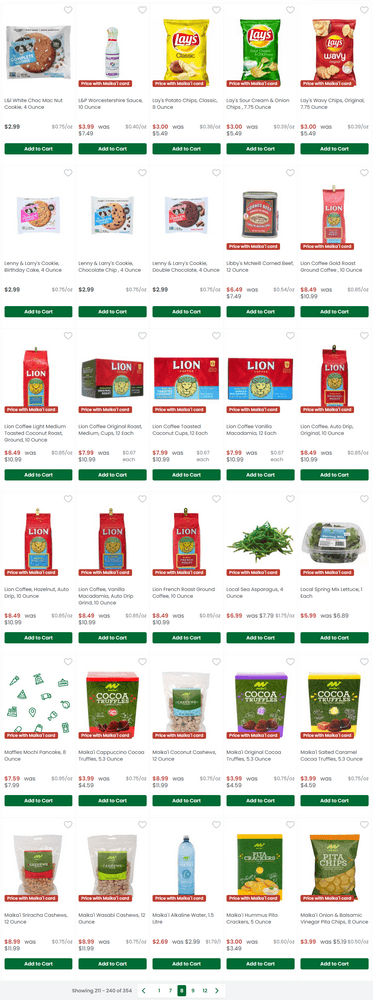This image displays a page from an online grocery shopping website, likely a platform similar to Instacart or Kroger, focused exclusively on food items. The page is structured into six rows, each containing five different packaged food products. Below each product is a green "Add to Cart" button, making it easy for users to select their desired items. Additionally, beneath each product's description, the price is clearly indicated. Visible products include popular brands such as Lay's potato chips and what appears to be Lion brand pasta, alongside other items like canned green beans, though the brand for these beans is not specified. At the bottom of the page, a navigation indicator shows that the user is viewing either page six or eight, with options to scroll left or right to browse additional pages.